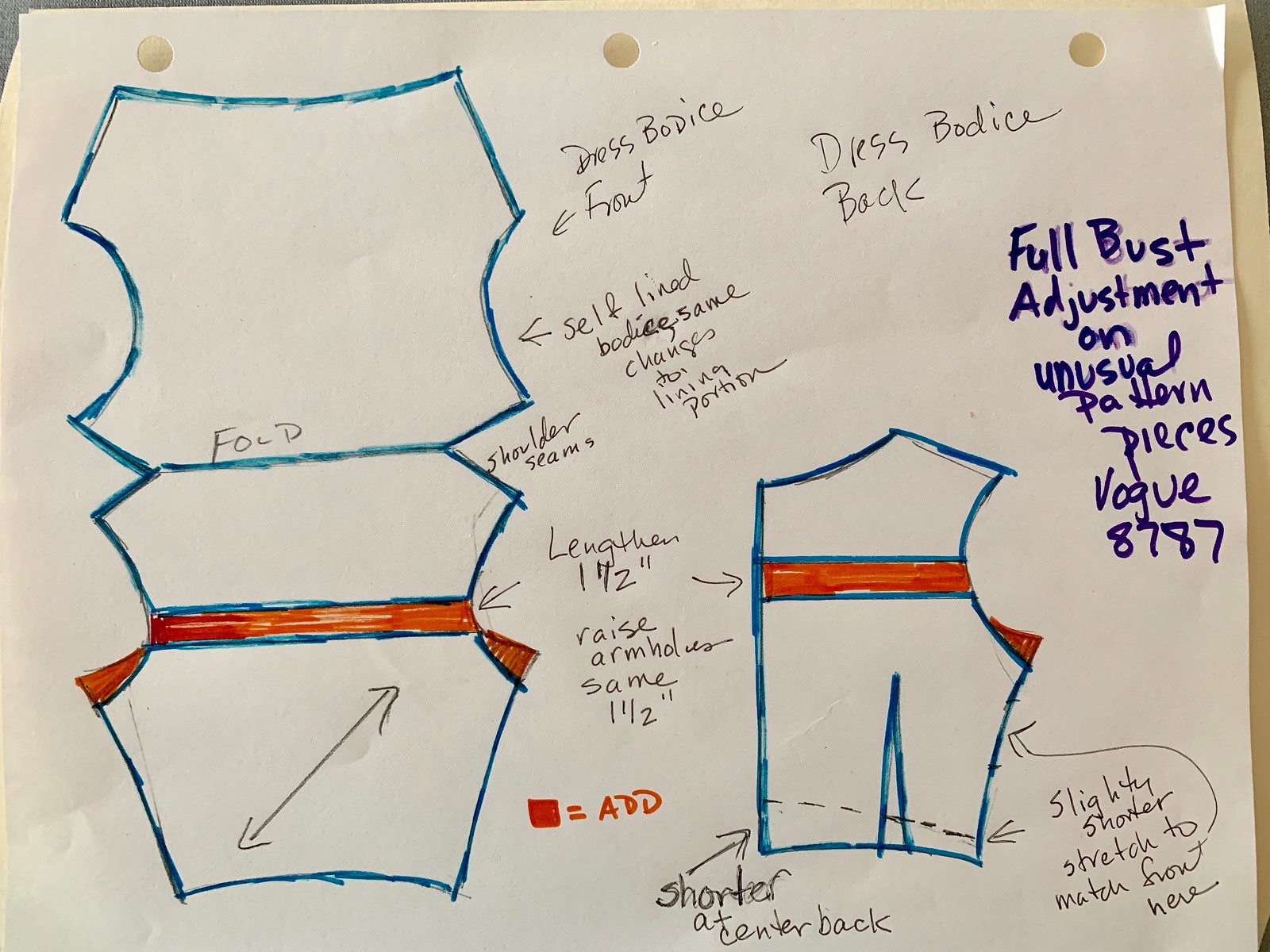The image is a rectangular photograph of a white piece of paper, pinned to a tan sheet underneath, both attached to a gray background with three tan thumbtacks. The white paper, oriented sideways with three hole punches across the top, features a detailed fashion design sketch marked in various colors.

At the top right, in dark navy or purple marker, the title "Full Bust Adjustment on Unusual Pattern Pieces, Vogue 8787" is prominently written. The paper is adorned with numerous diagrams in turquoise, blue, and orange, showcasing different pattern pieces with explanatory annotations. 

To the right of the paper, there are descriptions such as "dress bodice front" and "self-lined bodice," indicating specific parts of the design. Arrows point to different areas, illustrating folds and adjustments. One diagram highlights a fold symbol with an arrow stretching diagonally from the bottom left to the top right corner, labeled "you can fold it". 

Additional text details modifications like "shoulder seams" and "lengthen one and a half inches." There are directives such as "shorter at center back" with corresponding arrows and dotted lines indicating where to make cuts or adjustments. 

The sketch is a comprehensive and meticulous draft of a garment design, featuring instructional elements like “raised arm holders” and notes in black text, making it evident that this is an initial rough design of a complex fashion piece.